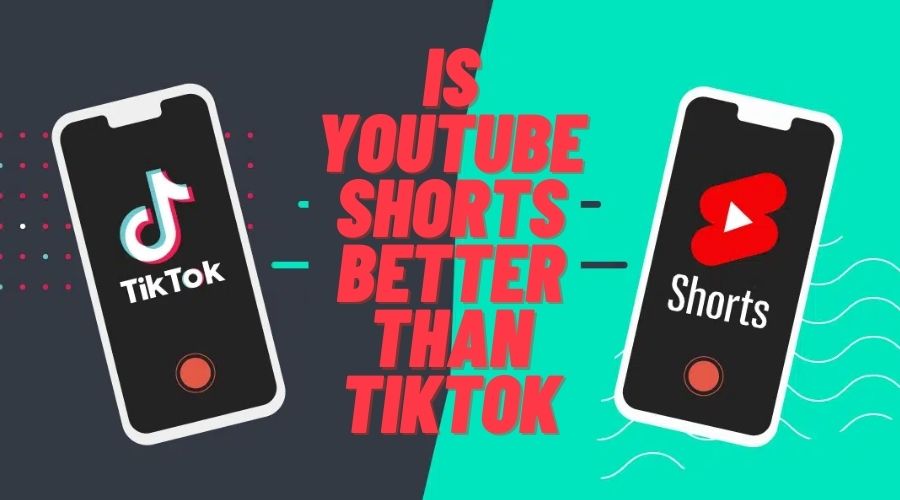The image features a divided background, with the left side colored in dark gray and the right side in aqua blue. On the left side, there is a small square adorned with red, white, and blue dots. This square houses a white telephone icon set against a black background, prominently displaying the TikTok insignia, which is white with blue and pink outlines. Below the logo, the text reads "TikTok." Adjacent to this are visual elements including a round red button and two small blue lines. The caption in bold red text asks, "Is YouTube Shorts Better Than TikTok?" 

On the right side of the image, another white telephone is displayed, this time bearing the red 'S' logo with a white triangle inside, identifying it as YouTube Shorts. The associated text reads "Shorts," and there is a red button below. The background here features subtle wave patterns in the aqua blue section. The question "Is YouTube Shorts Better Than TikTok?" is reiterated in the visual elements, inviting viewers to compare the two platforms.